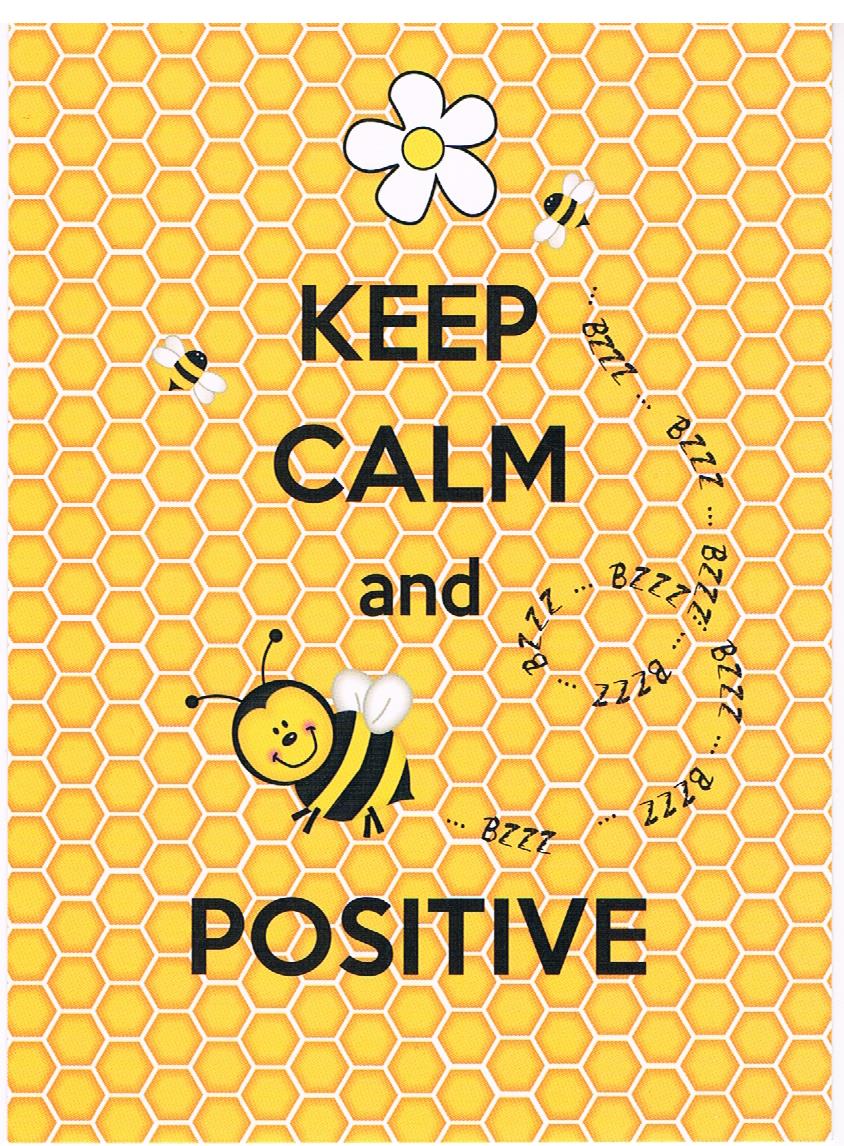This vertical rectangular poster features a vibrant honeycomb pattern in orange, outlined in white, forming a seamless background. At the top center, a white-petaled daisy with a yellow center sits prominently. Below the flower, in large bold black all-caps letters, the words "KEEP CALM" are displayed, followed by an image of a cheerful bumblebee with little white wings. Beneath the bee, the bold text continues with "AND POSITIVE." Two smaller bees, buzzing near the top-right of the poster, add a dynamic touch as their dotted flight paths twist and swirl around, spelling out "BZZZ." This artwork embodies an uplifting and artistic take on the classic "Keep Calm" motto, emphasizing positivity with its sunny hues and endearing bee characters.